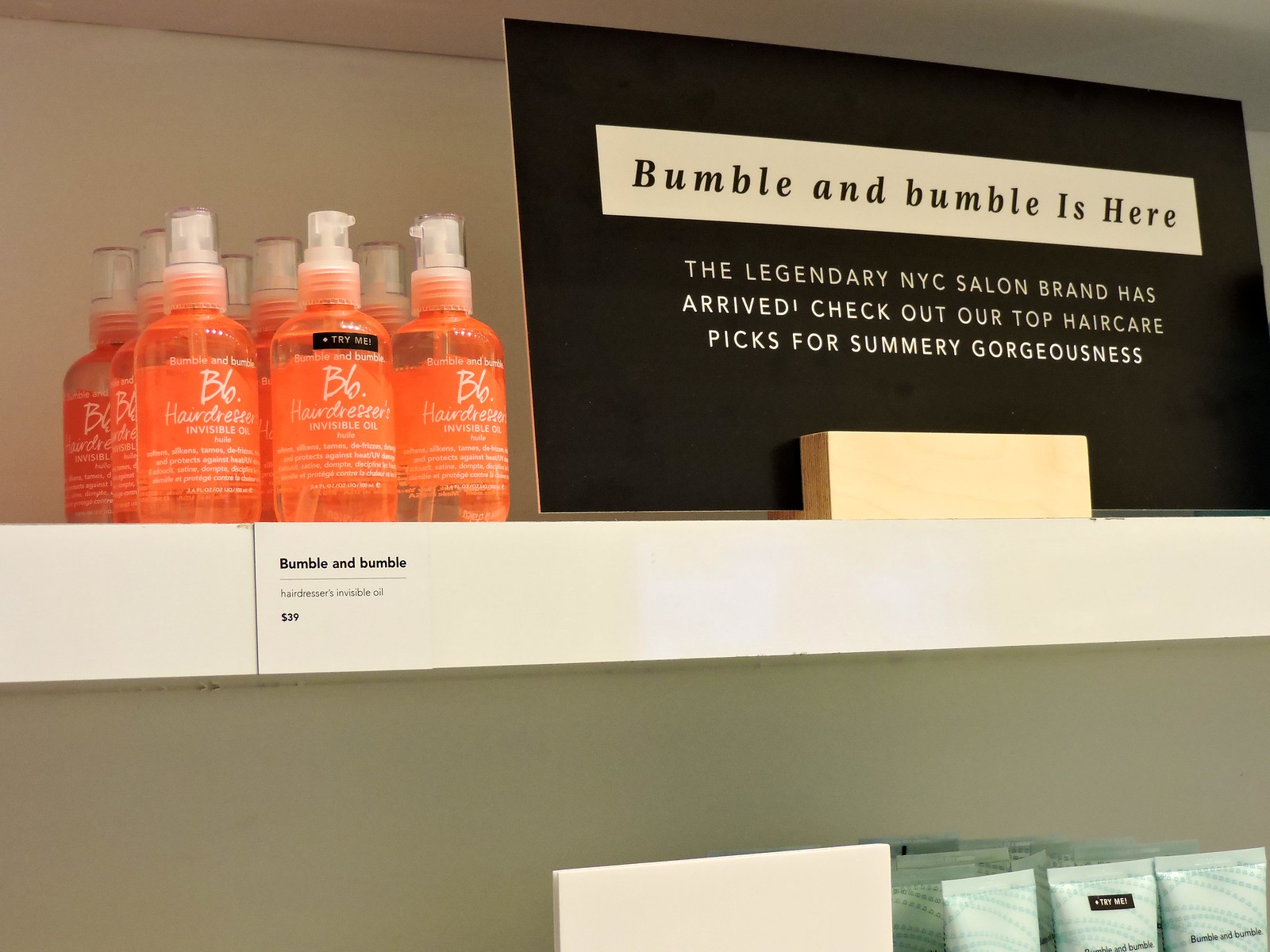This image captures a store shelf meticulously organized against a white backdrop. On the top left side of the shelf, there are nine neatly arranged orange and translucent bottles of Bumble and Bumble Hairdresser’s Invisible Oil. These bottles are displayed in three rows with white text that reads "BLO hairdresser’s invisible oil." The central bottle among them prominently features a black "Try Me" button and has a push pump at the top. Directly below the bottles, a black tag displays the product name "Bumble and Bumble Hairdresser's Invisible Oil" and the price "$39." 

To the right of the product display, a large black sign garners attention. At the top of the sign, within a small white rectangle, bold black text announces, "Bumble and Bumble is Here." Below this, on the black background, white text reads, "The legendary NYC salon brand has arrived. Check out our top hair care picks for summery gorgeousness." Beneath this sign, on the lower shelf, there are visible tops of other products, namely yellowy-green tubes and white squirt bottles adorned with blue dotted lines in their design.